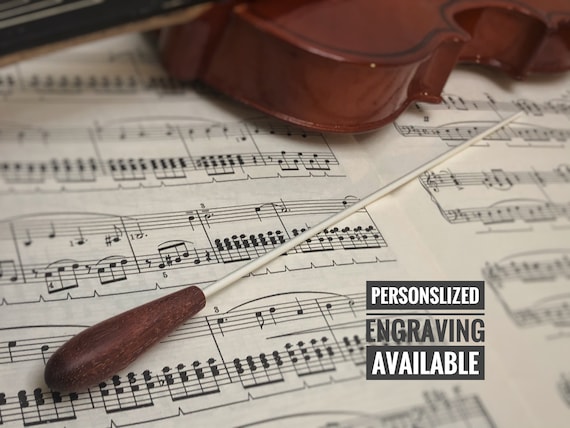The photograph captures a beautifully detailed scene of a music book open to several pages of sheet music. The left page showcases four visible rows of meticulously printed music notes, while the right page reveals three full rows and the beginning of a fourth. The sheet music is presented in black and white, providing a classic contrast. A portion of a wooden violin, notably its lower segment, lies atop the music book, with its strings extending to the left. Crossing the center of the image is a conductor's baton, distinguished by its elegant design with a brown wooden handle and a long, slender white rod that reaches toward the upper right corner. In the bottom right corner of the image, there is a colorful text message that says, "PERSONALIZED ENGRAVING AVAILABLE." The words "PERSONALIZED" and "AVAILABLE" are in white and all capitalized, while "ENGRAVING" is in black and also capitalized. This combination of musical elements and personalized message details creates a harmonious and visually appealing composition.